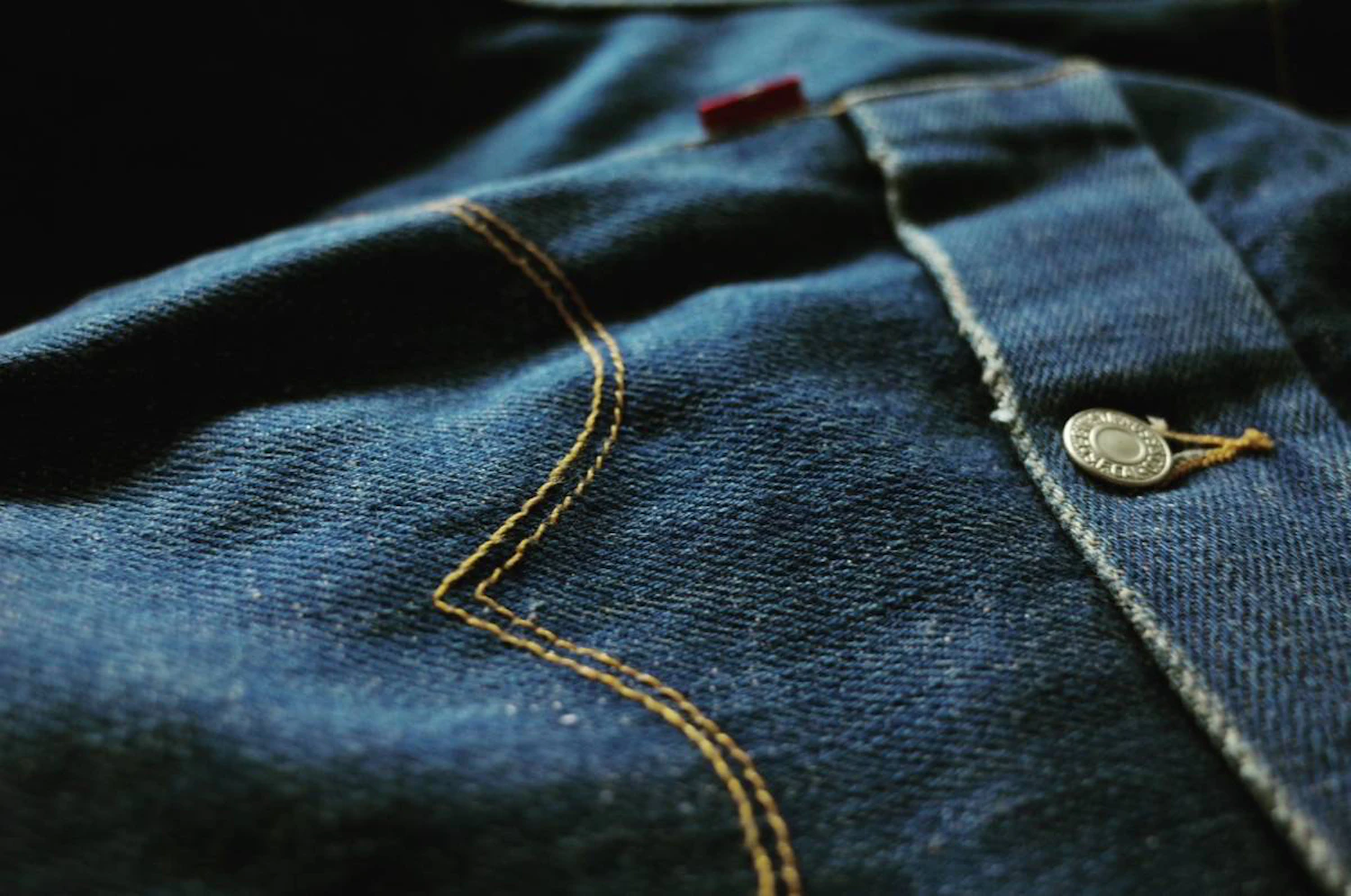This image captures a detailed close-up of a pair of dark blue jeans, focusing on a portion in the upper right quadrant. Dominating this section is a pocket secured with a silver button, which fastens through a buttonhole, keeping the flap of the pocket neatly closed. At the upper center of the frame, a distinctive red button adds a unique touch of color. Yellow thread stitching is prominently visible, starting from the center left, extending downward, and forming a V-shape towards the lower center. The area beneath the clasped button on the pocket is highlighted by a bordered white area, which starkly contrasts with the dark denim. Both the upper left and upper right corners of the image are shrouded in black, further emphasizing the intricate details and craftsmanship of the jeans, specifically the red button and the silver clasp.